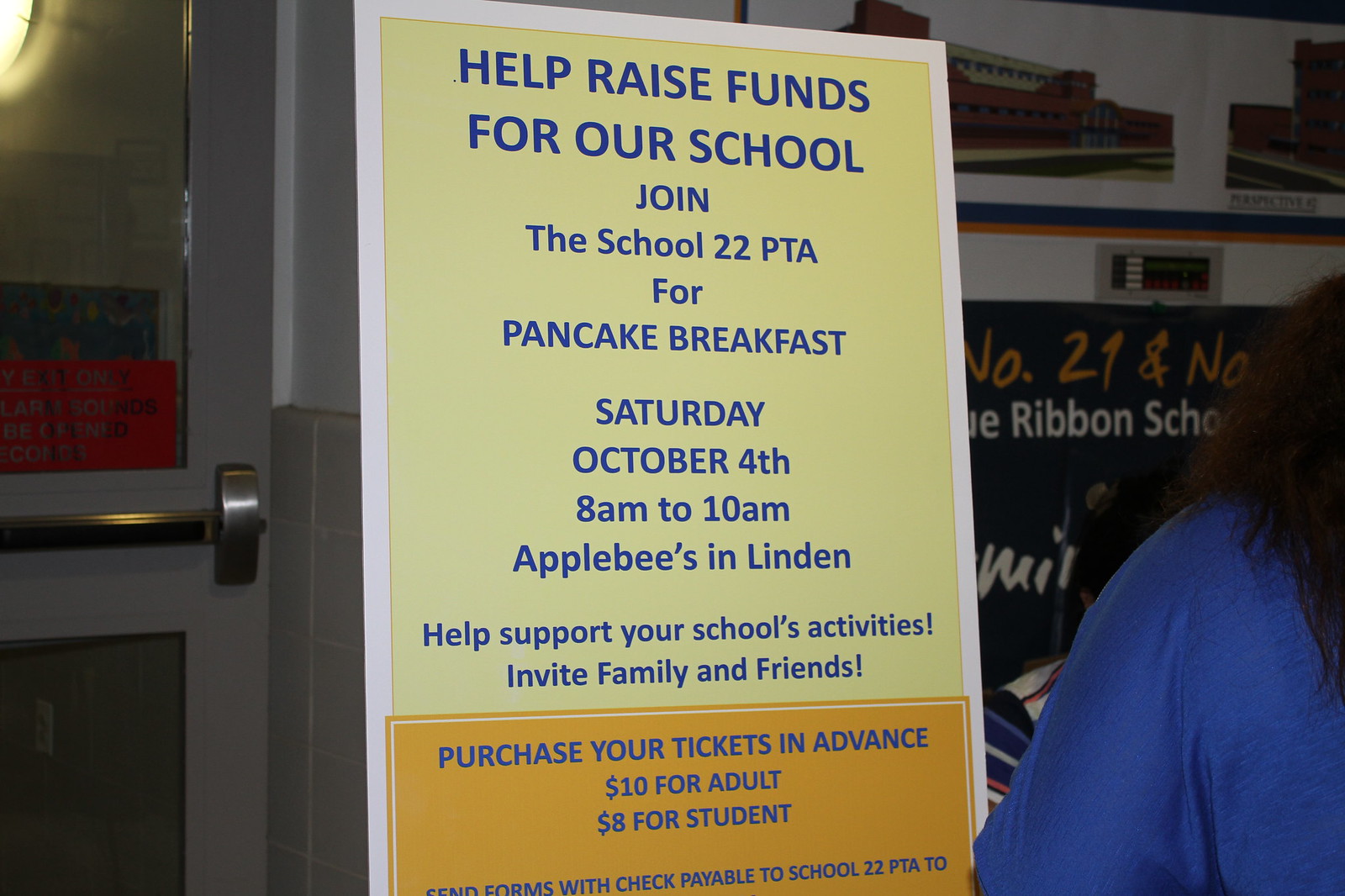The image shows a rectangular photograph likely taken inside a school, suggested by the setting and contents. Central in the photo is a large sign with a white border, which transitions from light yellow at the top to a golden orange at the bottom. The sign features blue text prominently reading: "HELP RAISE FUNDS FOR OUR SCHOOL." Below this, it continues: "Join the School 22 PTA for a Pancake Breakfast," with details including the event date, "Saturday, October 4th, 8 a.m. to 10 a.m.," and location, "Applebee's in Linden." The sign encourages community support with the line, "Help support your school's activities. Invite family and friends." In the golden orange section, it instructs: "Purchase your tickets in advance, $10 for adults, $8 for students. Send forms with a check payable to School 22 PTA to"—though the rest of the address is cut off. To the right, a partially visible person with long, dark brown hair and a bright blue shirt stands next to the sign. In the background, there are additional posters with unclear details and a door visible to the left. The setting includes wall decorations and gives a vibrant, community-centric feel.